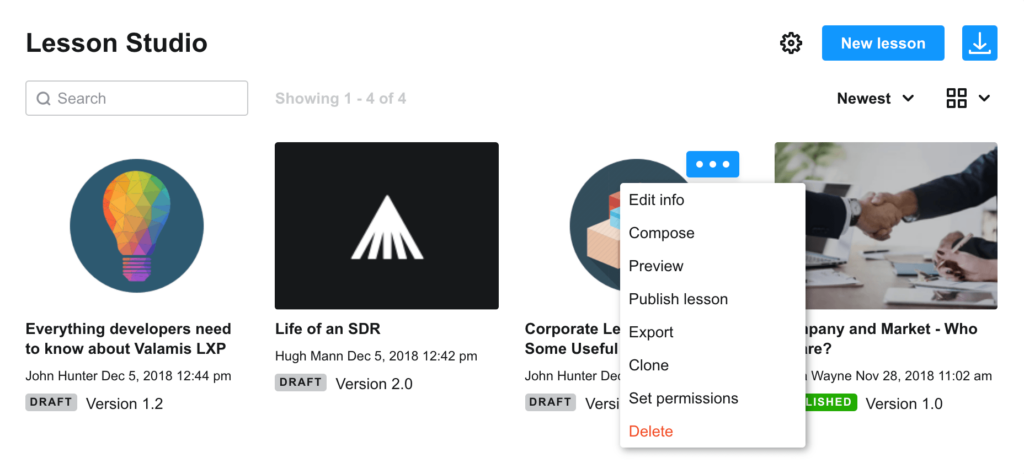The home page of Lesson Studio features a clean, white background. At the top left corner is the black text “Lesson Studio.” Below this text is a rectangular search window containing gray text with a magnifying glass icon, reading “Search.” Adjacent to the search window, it displays “Showing 1 through 4 of 4.”

In the upper right corner, there is a settings cog icon next to a blue rectangle with white text that says “New Lesson.” This is followed by a blue square featuring a directional arrow pointing down with a horizontal line beneath it. Immediately below this, it says “Newest” in black text, accompanied by a down-pointing arrow. Next are four small squares forming a larger square pattern, alongside a dropdown menu icon with a directional arrow pointing down.

Moving further down on the far left, there is a circle with a rainbow-colored light bulb icon. Below this, it reads “Everything Developers Need to Know About Volumis LXP” by John Hunter, dated December 5, 2018, at 12:44 PM, followed by the text “Draft Version 1.2.”

To the right of this is a black square featuring a white mountain icon. Below, it says “Life of an SDR” authored by Hugh Mann, dated December 5, 2018, at 12:42 PM, with the text “Draft Version 2.0.”

Next to this is a circle surrounded by some boxes with the text “Corporate Le, Some Useful.” Below it, it reads “John Hunter” and “Draft.” Superimposed over this section is a white rectangle with black text options: “Edit Info,” “Compose,” “Preview,” “Publish Lesson,” “Export,” “Clone,” and “Set Permissions.” At the bottom in red text, it says “Delete.”

Beside this section is an image of two men in business jackets shaking hands, captioned “Company and Market, Who, Where” by Wayne, dated November 22, 2018, at 11:02 AM, with the text “Version 1.0.”